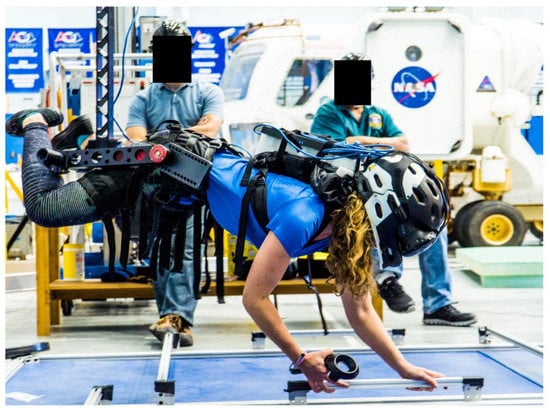The photograph captures a woman engaged in a detailed training simulation, possibly for astronaut training, set in an indoor area with NASA branding prominently displayed. She is dressed in a short-sleeved blue shirt, tight gray leggings, and black shoes. Her head is encased in a dual-tone virtual reality headset, black in the front and white in the back, and she holds a virtual reality controller. 

Her entire form is supported by a complex metal armature at her waist, keeping her torso parallel to the ground. Leaning forward, she grips handles on a blue, door-like structure on the floor, suggesting a low-gravity simulation environment. 

In the background, two men with folded arms and obscured faces observe her closely, seemingly involved in the simulation process. To the top right, a white vehicle with the iconic NASA logo—a blue circle adorned with white letters, a red streak, and a half-circle—adds to the authenticity of the scene. A yellow cart is also visible, adding an additional element to the intricate setup.